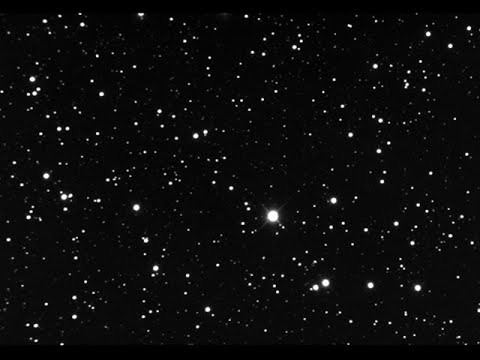The image is a slightly rectangular shot of space, featuring a predominantly black background speckled with hundreds of white dots representing stars of various sizes. Among these stars, some are faint and small, while others are brighter and more prominent. Notably, towards the center of the image and slightly down and to the right, there is a particularly bright and large circular star that stands out. This central star is characterized by rays of light emanating from it, reminiscent of the North Star. As the gaze moves towards the bottom of the image, the stars become progressively fainter and smaller, creating a sense of depth and vastness in this telescopic photo of the night sky.